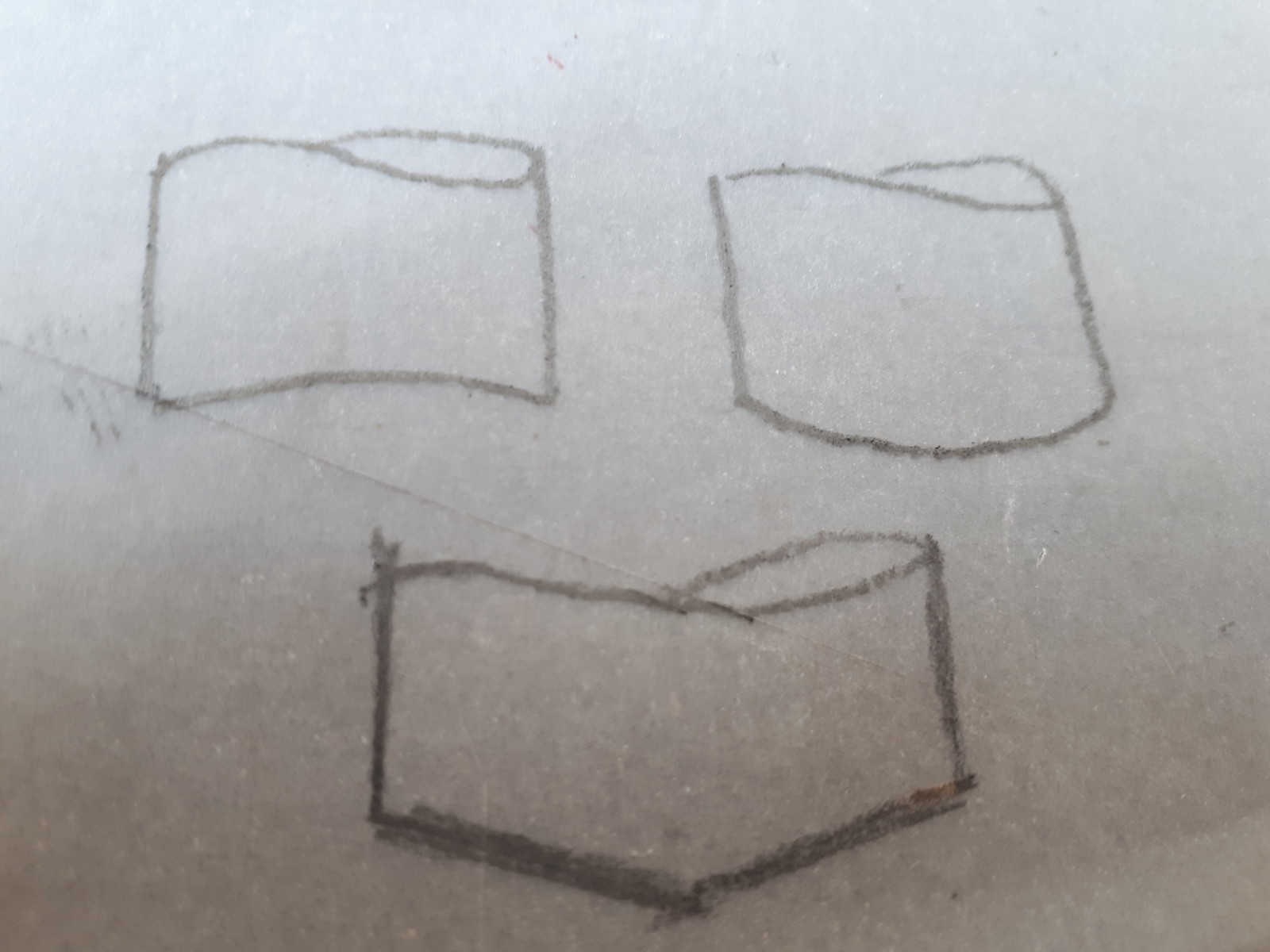This image appears to be a high-resolution scan or photograph of a digitally illustrated artwork, abstract in nature. The illustration, which has been cropped and edited, showcases three distinct objects resembling marshmallows. These objects are set against a textured piece of white paper, noticeably rougher than standard paper, with visible inclusions of different shades of white and gray. A prominent crease runs through the center of the paper, accompanied by faint black lines on the middle left, suggesting possible ink smudges. 

The three objects are arranged as follows: The top left object has a rounded bottom, bulging upwards, and features a loop on the top right, adding a 3D illusion. The top right object mirrors the first but with a rounded bottom curving downwards. The third object is centrally placed below the first two, forming a downward-facing triangular shape, and also includes the characteristic loop at the top right. The overall minimalist background further accentuates these unique shapes, rendering a visually compelling abstract composition.